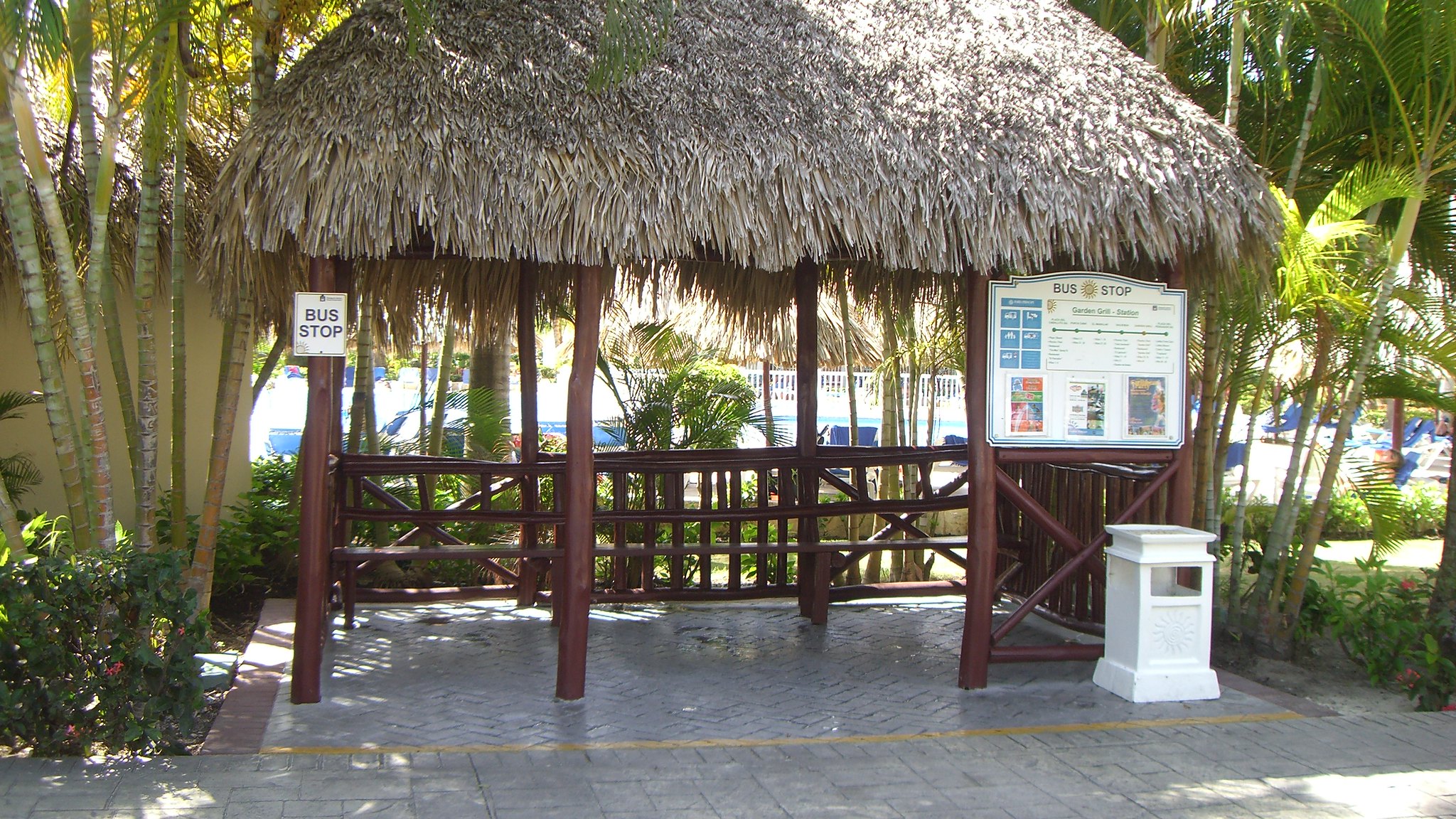A detailed photograph captures a tropical bus stop situated outside on a bright, sunny day. The bus stop, centrally framed, features a tall, triangular roof made of beige, dried leaves reminiscent of a tiki hut. Supported by reddish-brown wooden posts that evoke the texture of tree trunks, the structure includes finer logs forming a low railing around the back, complementing a matching low bench. Prominently, there are two bus stop signs: a smaller one on the leftmost pole and a larger one on the right that likely lists the routes. Directly below the larger sign is a white, windowed trash can. The background is adorned with towering palm trees and dense, flowering shrubs, suggesting the ambiance of a resort, further emphasized by a glimpse of a pool. The sunny conditions cast distinct shadows, particularly illuminating the right side of the bus stop's leafy roof. The entire setting is built upon a grey, brick-paved sidewalk, enhancing the overall tropical feel of the scene.